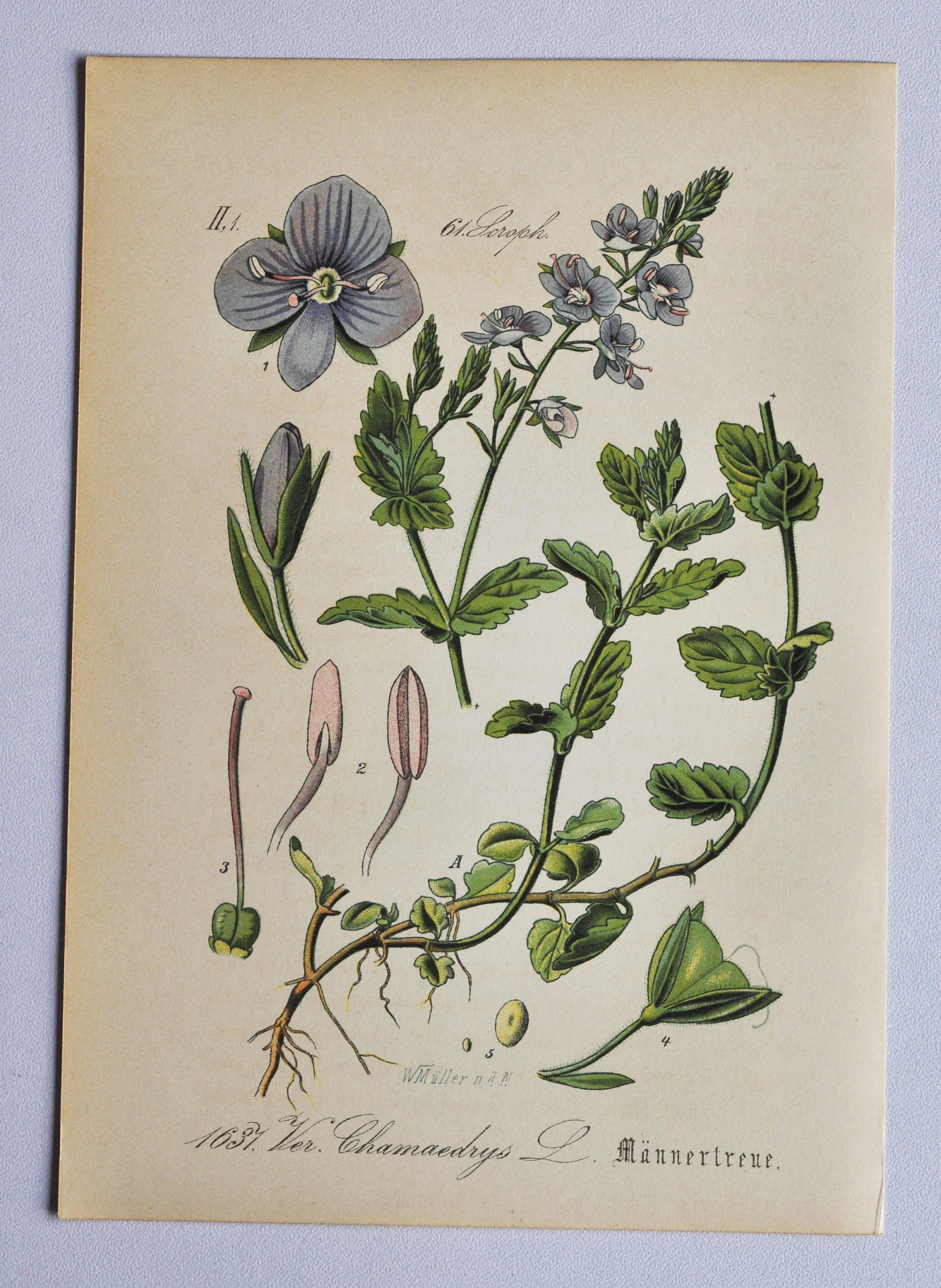The image depicts an aged, yellowed page from an old botanical book mounted on a light blue surface. The page features a detailed, colored illustration of a plant, showing various stages of its growth and parts. The plant illustration includes green stems with sharp and teardrop-shaped leaves, as well as a series of flowers and buds. The flowers, positioned at the top of the plant, have four petals each, shaded in a dark grayish-blue with dark blue stripes, and surrounded by white bulbs. Some flowers are shown in the budding stage with pink and white-gray stems. The drawing is comprehensive, showing the plant from its seedling stage to its full bloom, numbered to indicate different growth phases. Below the illustration, there is cursive text in black ink which partially reads "1631." The page overall has text that includes "ver 1631 ver gematris L" and other legible and illegible cursive scripts. The detailed depiction, along with labeled stages and meticulous plant features, suggests a scientific and educational purpose, highlighting the botanical interest of the era.